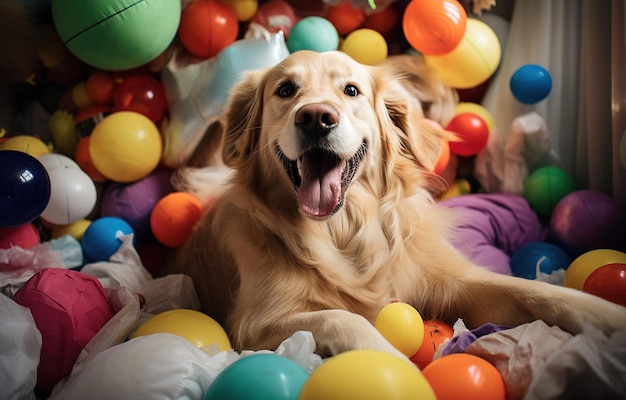In this cheerful photograph, a light-colored, possibly golden, long-haired dog is comfortably laying down with its front paws stretched out in front of it. The setting is vibrant, as the canine is surrounded by a multitude of colorful balloons in shades of orange, red, yellow, blue, lavender, and pink. The dog reclines on a plush and fluffed-up pad, looking undeniably content and relaxed. In the backdrop, a set of curtains is partially visible, suggesting that the scene is set in a cozy living room. This delightful scene conveys a sense of joy and tranquility, making one wish to reach out and pet the happy dog amidst its festive surroundings.